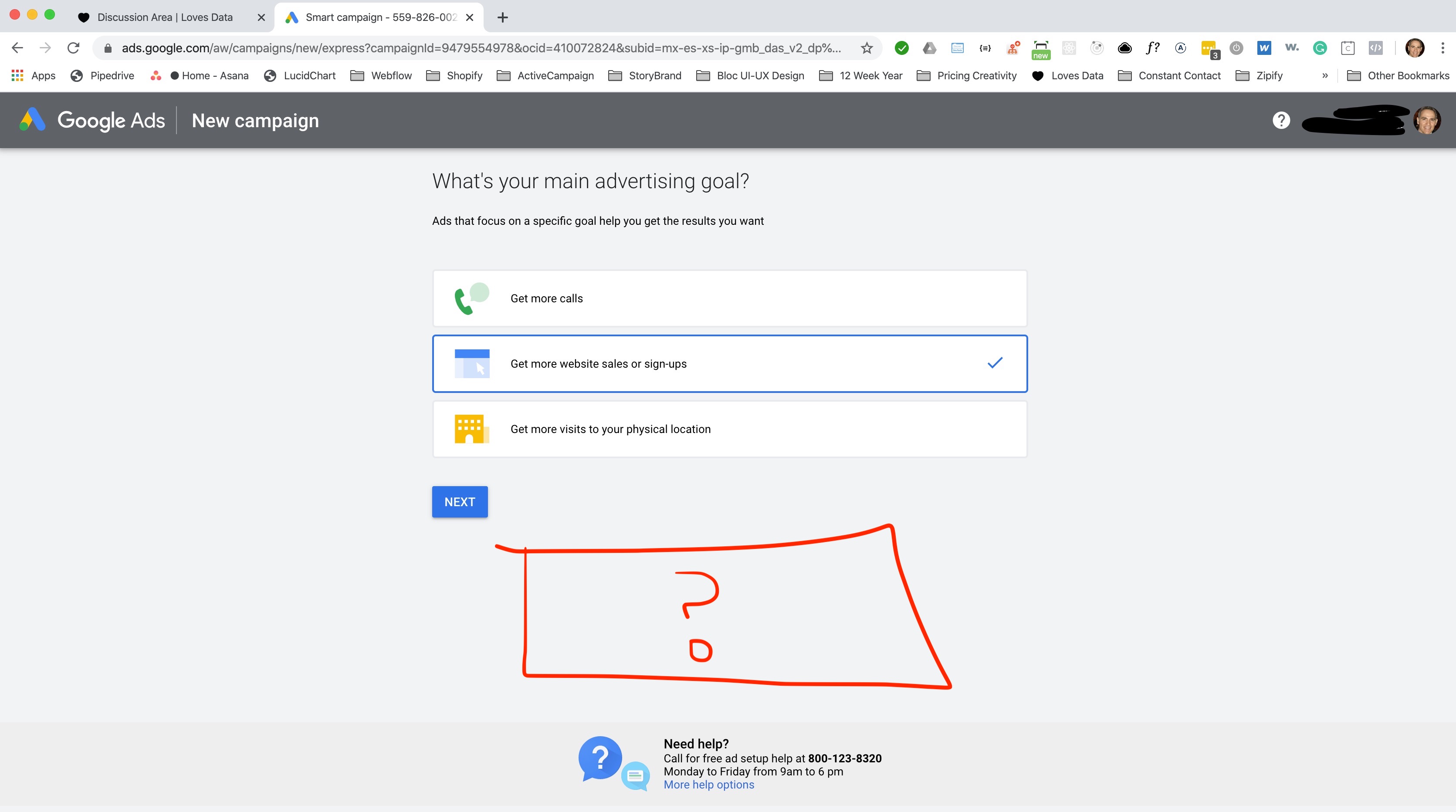In the image, various elements are vividly highlighted in red, yellow, and green colors. The central focus appears to be on a discussion area, symbolizing a place where data enthusiasts gather. Additionally, themes relating to a smart campaign are visible, with the number 559-866-008 potentially hinting at a contact point or a significant detail. The image is dominated by references to Google search, emphasizing repeated searches, which might suggest intensive research or the importance of finding information online. Overall, the image encapsulates the intersection of data love, campaign strategy, and the pursuit of knowledge through incessant online searches.